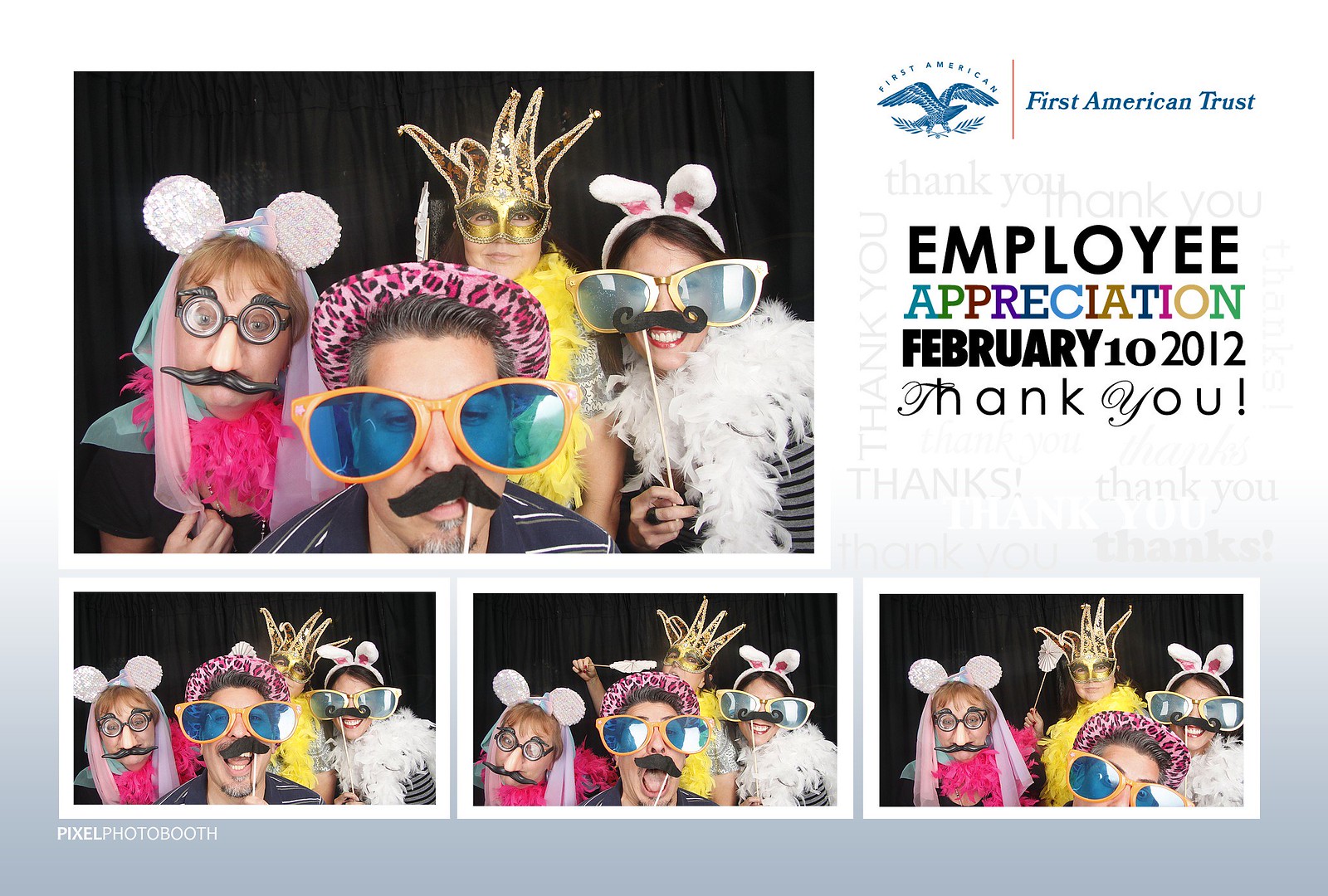The image captures a lively scene from an event, showcased through a series of four photographs against a gradient background that transitions from gray at the bottom to white at the top. In the top right corner, the identity of the event is made clear by a detailed text alongside a logo. The logo features a stylized blue cartoon eagle facing right, clutching two leaves in its claws, with the words "First Americans" above it. Adjacent to this logo, in blue text, reads "First American Trust." Below, the text commemorates "Employee Appreciation, February 10, 2012. Thank You." The word "Appreciation" stands out vividly with each letter in a different color: blue, green, purple, black, blue, and so forth.

The photographs prominently display four people engaged in a festive, costume-themed activity. The top left photo shows three people in the foreground and one in the background, all donning comical and elaborate costumes that include oversized sunglasses, colorful mustaches, bunny ears, a feathered crown, and vibrant boas in yellow and white. The participants' outfits are further enhanced with accessories like leopard print pants and hats, contributing to the playful atmosphere. The backdrop of these images is a set of black drapes, which helps highlight the costumes.

Below this primary image, three additional variations of the same setting capture the same group of four individuals in different playful poses, maintaining the same headgear and attire. Each photograph focuses on their head and shoulders, emphasizing their spirited and silly expressions. Overall, the sequence of photographs captures the essence of the celebration and camaraderie at the event, set against a thoughtfully designed backdrop and detailed with event-specific text and logos.